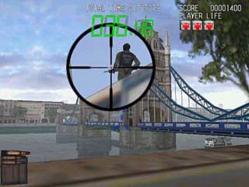The image appears to be a still from a first-person shooter (FPS) video game. At the center, there is a black circular crosshair with four short lines radiating towards the middle, indicating the player's aim. The scope is focused on the back of a man wearing a gray shirt, who is holding a gun. This scene takes place on a large stone bridge with blue sections, spanning over a river that reflects the structure above. 

In the background, there are gray buildings and a tree in the top right corner. The sky transitions from blue at the top to whitish towards the horizon. The game interface (UI) is visible at the top of the screen, with white elements and green numerical indicators, along with three red shapes on the top right. In the lower left corner, there appears to be an object resembling a garbage can.